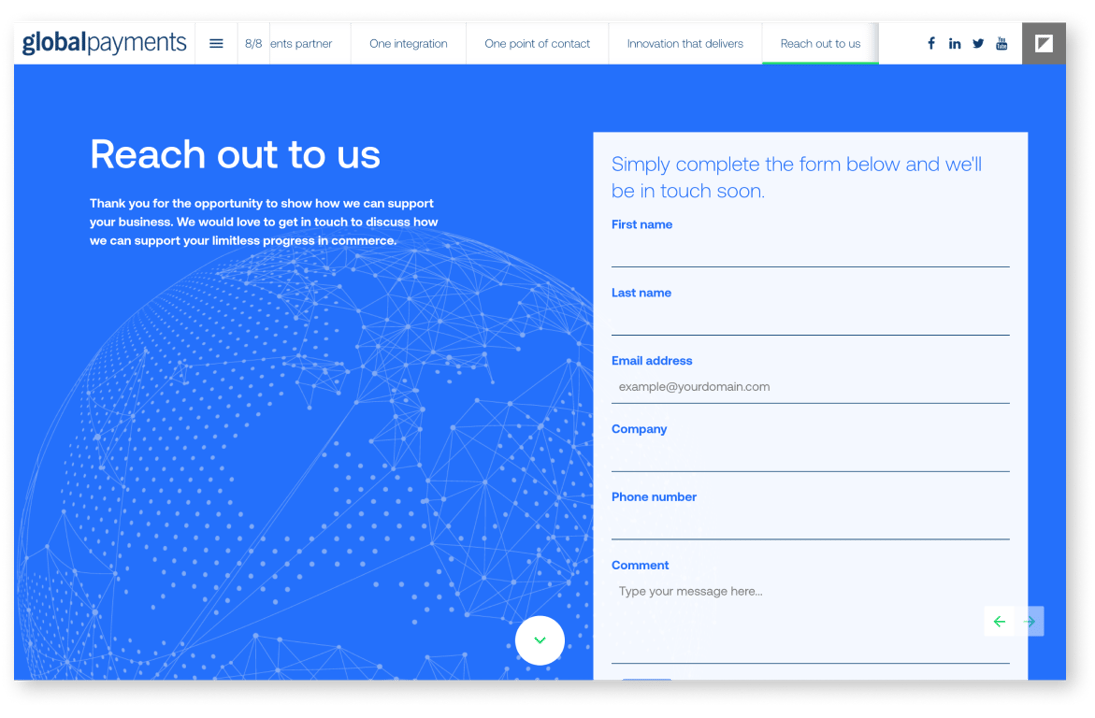Screenshot of the Global Payments website showcasing its user interface and contact form. In the upper right corner, the website's name, "Global Payments," is displayed in dark blue font against a white header. Adjacent to the website name is a hamburger menu icon and a horizontal menu strip featuring navigation options such as "One integration," "One point of contact," "Innovation that drives," and "Reach out to us." The currently selected tab, "Reach out to us," is highlighted with a green stripe at the bottom.

Dominating the main portion of the website is a blue background illustrating a globe-like sphere interconnected with numerous dots and lines, symbolizing global networks and connections. Overlaid in white text are the words: "Reach out to us," followed by a welcoming message: "Thank you for the opportunity to show you how we can support your business."

Below this text, there is a prominent white rectangle containing a contact form. The form includes blue text instructing users: "Simply complete the form below and we'll be in touch soon," and provides fields for the user to enter their information.